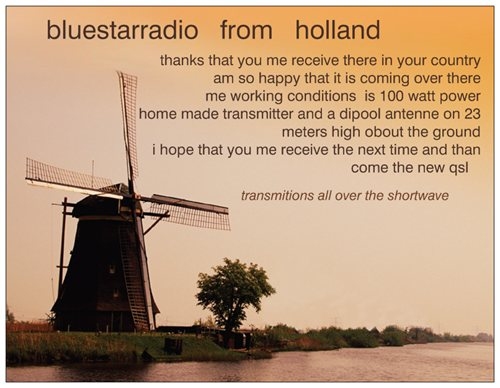The image features a sepia-toned, landscape-oriented photograph with an orange-tinted background. Dominating the top portion, black text reads "Blue Star Radio from Holland," followed by a smaller, right-aligned paragraph. The message expresses gratitude for the reception of the broadcast in other countries, mentioning a homemade transmitter with 100-watt power and a dipole antenna positioned 23 meters above the ground. It also anticipates future QSL transmissions over shortwave radio. The bottom left corner of the image showcases a vintage Dutch windmill with a large conical roof and four substantial propellers extending in all directions. A small tree stands beside the windmill, and both are positioned on a spit of land that overlooks a body of water, adding to the scenic charm of the composition.